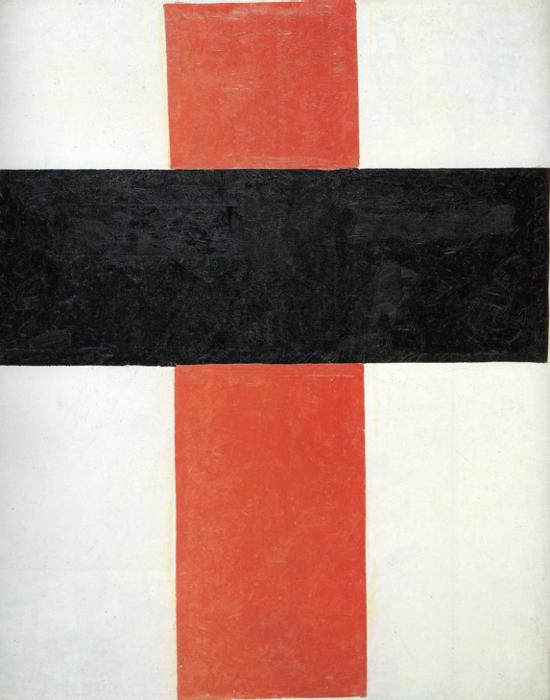The artwork depicts a semi-simplistic image on a white or off-white background, likely a piece of paper. Central to the composition is a vertical block of rose-red color that spans one-third of the width and extends from the top to the bottom of the page. This vertical line slightly inclines to the left as it descends, giving it an uneven, hand-painted appearance. A black horizontal block intersects this red vertical line three-quarters of the way up the page, forming a cross-like structure. The arrangement of the colors is somewhat opaque and muddy, with various shades of red and black suggesting layers of paint that have been scraped or overlaid, rather than a single solid color. This gives the piece a textural, painterly quality. The intersection of the lines divides the white background into four asymmetrical sections, reminiscent of certain flag designs, yet distinctly non-symmetrical and unique in its execution.